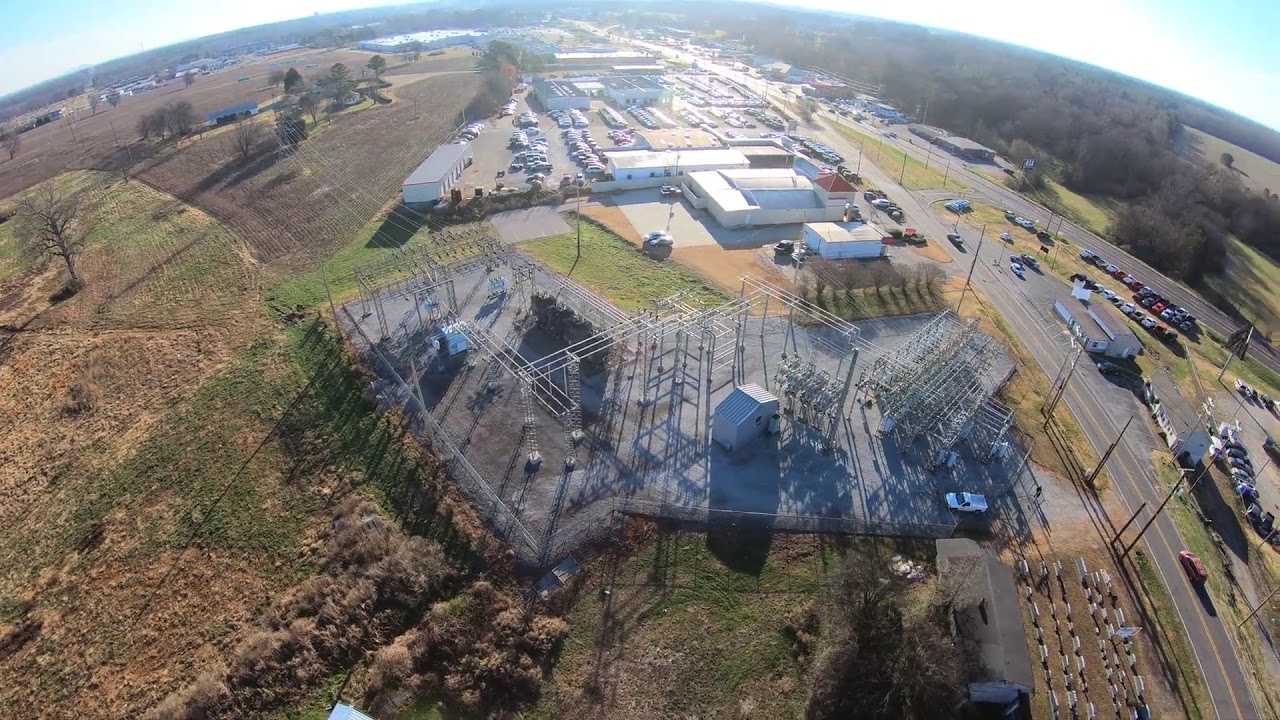The image is a detailed aerial view, likely taken from a drone, capturing a diverse landscape in vibrant color. The central focus is an electrical substation plant, situated on a gray concrete surface formed by two intersecting rectangles, and equipped with overhead wiring and a small shed at its core. A network of metal poles and electric lines extends out from this industrial area, connecting to other parts of what appears to be a city or possibly a college campus. This complex is surrounded by smaller white commercial buildings featuring parking lots crowded with cars. On the right side of the image, two streets converge, showing a mix of moving and parked vehicles, with the roads leading toward the horizon. The left side of the photograph reveals a patchwork of green grass and brown dirt, punctuated by a few small trees and bushes, reflecting a mix of farmland and possibly burnt-out areas. The entire scene is shown in a convex perspective, creating a slight curvature that emphasizes the horizon, contributing to a sense of global context. The image, characterized by photographic realism, captures the blend of urban infrastructure and natural landscape from a bird’s-eye view.